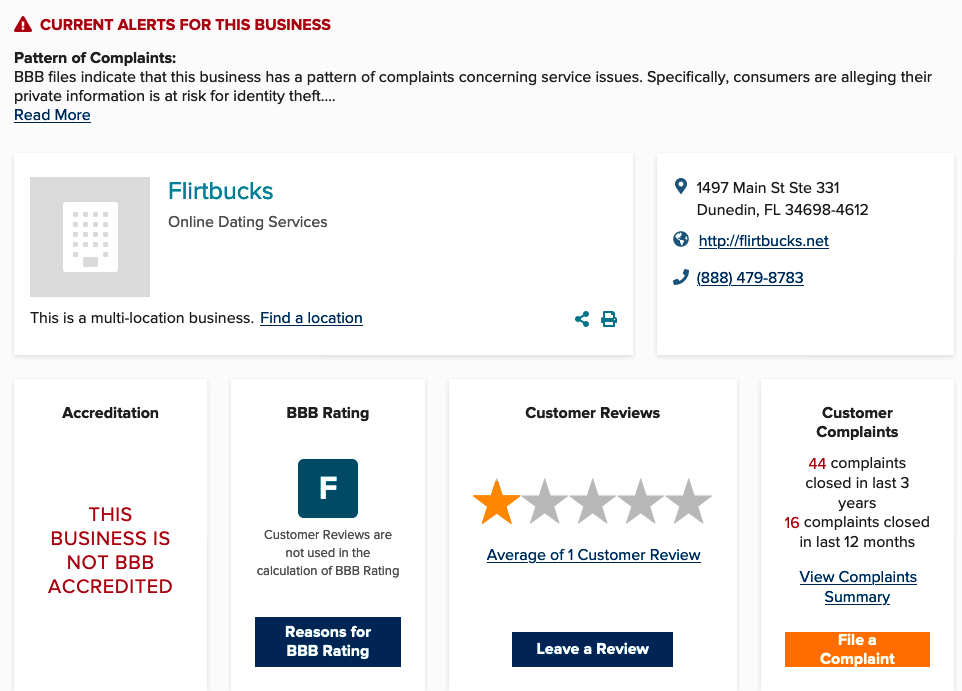In the upper left-hand corner of the image, there is a red notification that reads "Current Alerts for This Business." Below this, a highlighted section outlines a pattern of complaints. The Better Business Bureau (BBB) files indicate that this business has recurring issues concerning service problems, specifically noting that consumers are alleging their private information is at risk for identity theft.

Further down, the image is divided into two sections or squares. The first section features the text "Flirt Bucks" in blue, followed by a grey subtitle that reads "Online Dating Services." To the right, the second section displays an address: 

"1497 Main Street #331,
Dunedin, Florida 34698-4612."

It also includes a website URL: "flirtbucks.net."

Below these sections is a detailed four-part description:

1. **Accreditation:** This business is not BBB accredited.
2. **BBB Rating:** The business has been assigned an "F" rating.
3. **Customer Reviews:** The average rating from customers is one star.
4. **Customer Complaints:** There have been 44 complaints closed in the last three years.

Additionally, each of the last three sections features clickable buttons:

- Under "BBB Rating," there is a button labeled "Reasons for BBB Ratings."
- Under "Customer Reviews," there is a button for users to "Leave a Review."
- Under "Customer Complaints," there is an orange button with white text labeled "File a Complaint."

The image provides a thorough breakdown of critical information regarding the business’s service quality and customer satisfaction.